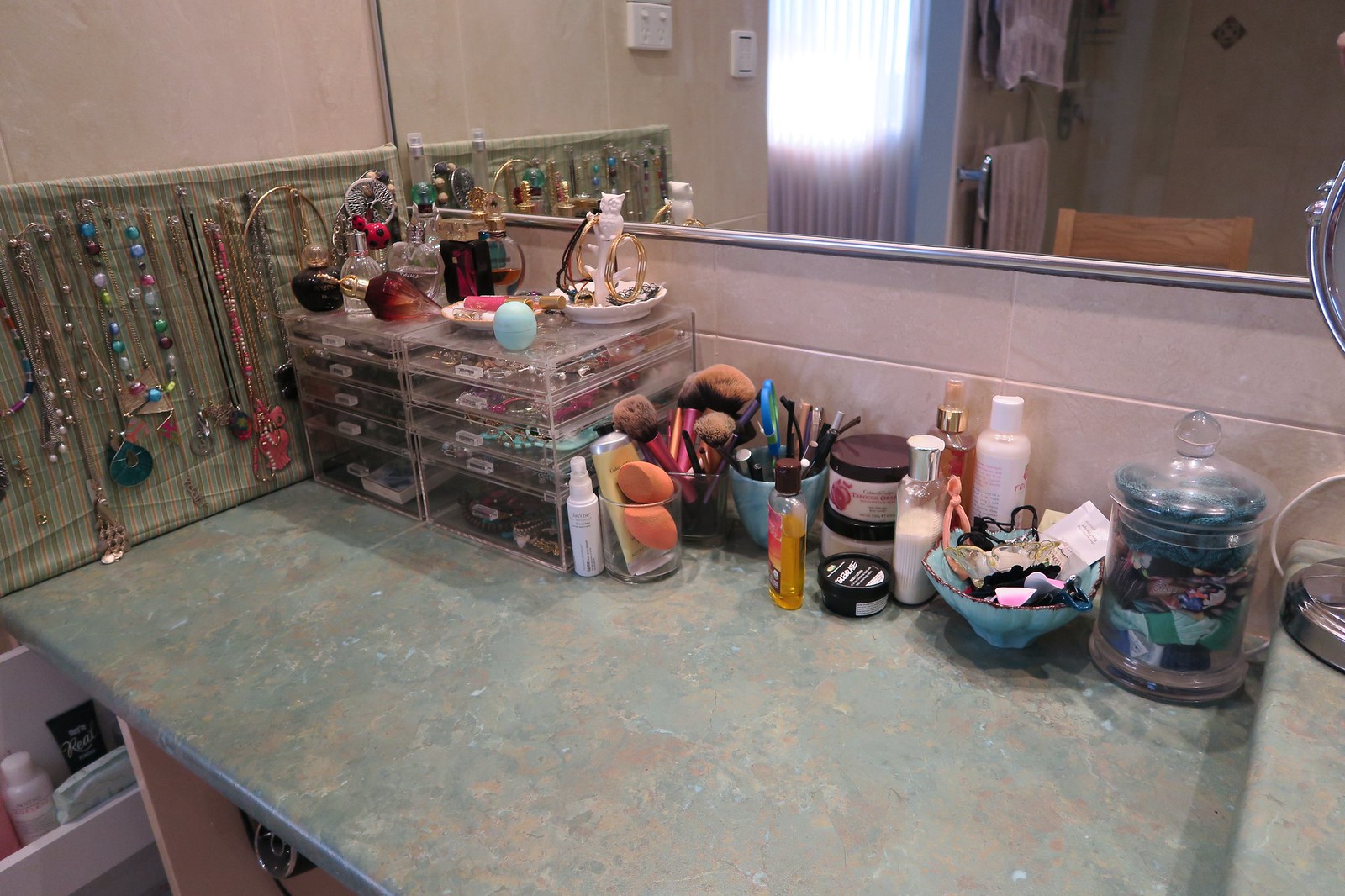This image captures the detailed interior of a bathroom. The main focus is a large countertop predominantly green in color, speckled with bits of brown and white. The beige-pink wall backdrop adds warmth to the setting. Positioned above the countertop is a sizable mirror that reflects a window with blinds, two towels neatly hung on racks, and a brown chair in the background.

The countertop itself is cluttered with various items. On the left side of the wall, there is a rack holding numerous necklaces. Below this, transparent containers with drawers store an assortment of jewelry, with even more jewelry pieces displayed on top. Moving to the right, there is an array of makeup products, including puff applicators, brushes, and scissors. There is also a mug organizing additional items, accompanied by various creams, hair ties, and other beauty products.

At the far right edge of the image, part of another mirror is barely visible. In the bottom left corner, more creams, including a black and a white tub, are arranged on a small white rack, completing the detailed snapshot of this personal space.